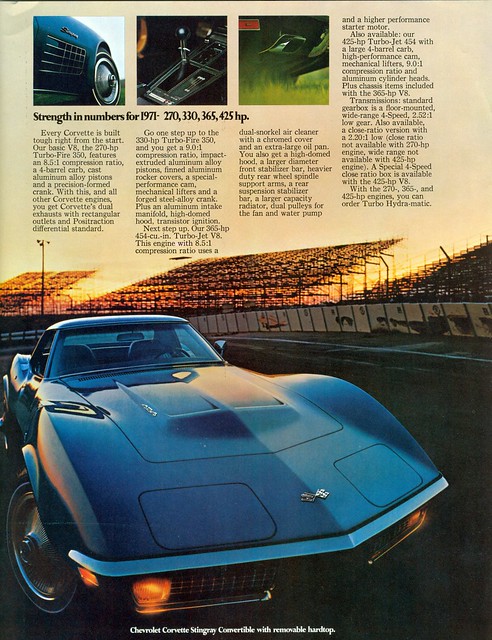The image appears to be a page from a vintage magazine featuring a detailed advertisement for a Chevrolet Corvette Stingray Convertible with a Removable Hardtop. The primary focus of the image is a striking blue Corvette prominently displayed in the lower section, photographed at a slight angle to highlight its sleek design. The background reveals an empty stadium with bleacher-style seating, suggesting the setting is a racetrack or similar venue. The caption at the bottom reads "Chevrolet Corvette Stingray Convertible with Removable Hardtop" in clear white lettering.

The top portion of the magazine page includes an article titled "Strength in Numbers for 1971," boasting engine power options ranging from 270 to 425 horsepower. Accompanying the text are three smaller images showcasing specific details of the Corvette: the front fender and wheel, the center console with the shifting knob, and an indistinct third image, partially obscured by grass. The overall layout combines these visual elements with several paragraphs of descriptive text, enhancing the advertisement's nostalgic and informative appeal.